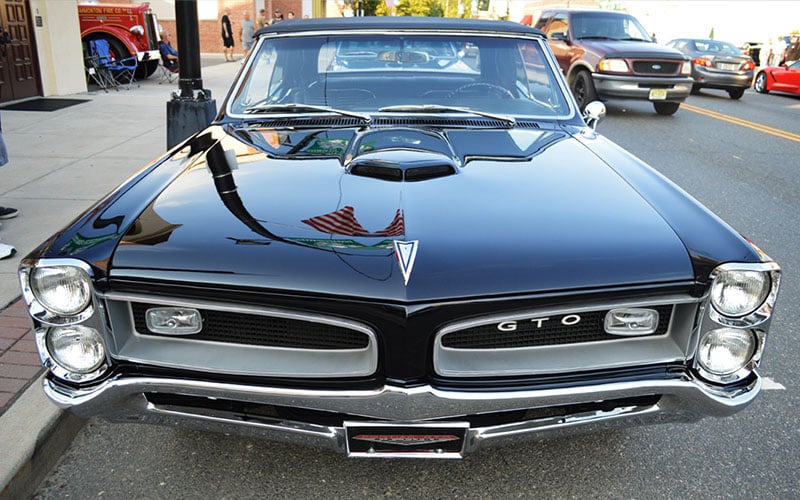The image features a gleaming black vintage car, likely a GTO model judging by the emblem prominently displayed on its distinctive two-part front grille. The grille, adorned with the "GTO" logo in white letters, is flanked by an ornate chrome bumper with pairs of headlights on either side. The car's polished exterior underscores its probable status as a luxury vehicle in its era. The hood carries a noteworthy design element: a downward-pointing triangular shape outlined by a black line, adding to its classic appeal. 

Through the car's exceptionally clean windows, details of the interior, including the steering wheel, are visible. The vehicle is parked on a street marked by a yellow line, surrounded by other vehicles such as a red truck, a red car, and a gray car. Nearby, a lamppost stands by the sidewalk, which is furnished with some blue chairs next to a building with brown doors. In the background, a fire truck is partially visible.

The scene is lively, with several people congregating and conversing. The individuals are dressed in various shades of gray and black, with some wearing hats. The setting is further enhanced by the presence of trees, which provide a natural backdrop to this vibrant urban tableau.